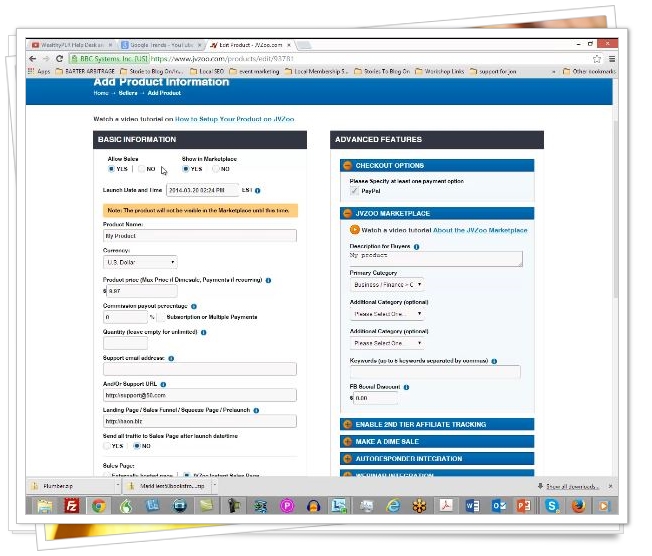This image depicts a blurry screenshot of a Google-hosted website, making the web address unreadable. The webpage in focus appears to be a product information setup interface, identifiable by the heading "Add Product Information." Three browser tabs are open at the top, with one of them being a YouTube video.

The visible layout of the webpage shows three primary tabs labeled "Home," "Before," and "Add." Underneath the main header, there's a section that reads "Watch a video tutorial on how to set up your products," suggesting instructional content is available for users. 

On the right side of the webpage, there's a section titled "Advanced Features," and on the left, one labeled "Basic Information." Both sections contain multiple text boxes designed for users to input various details. Although the image is blurred, the overall structure and layout of the website interface are discernible.